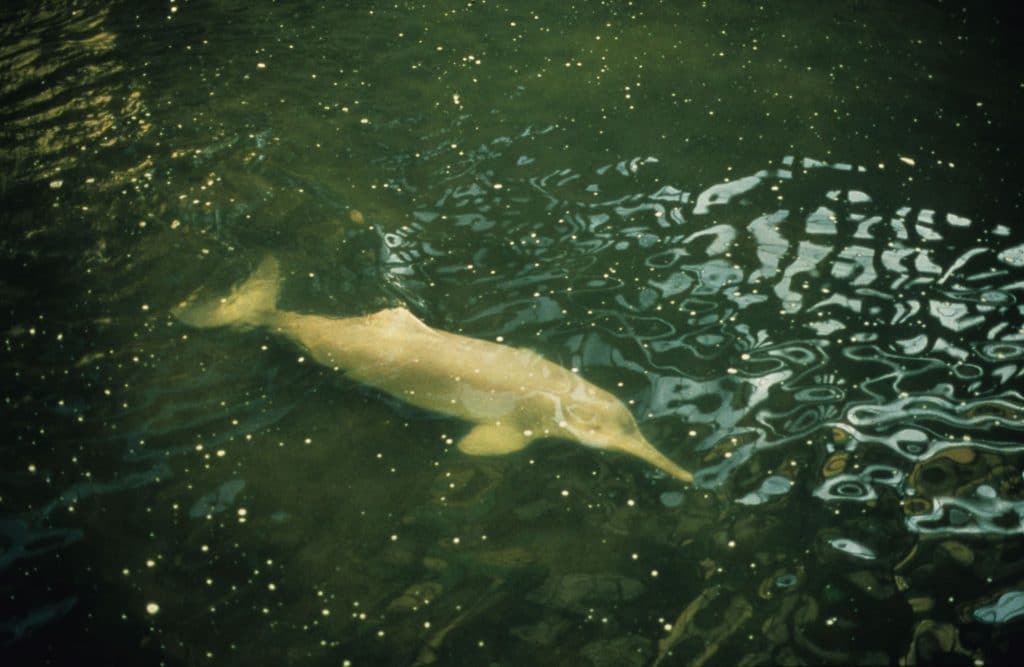The photograph captures a slender, fish-like sea creature swimming in dark, brackish waters, which exhibit varying shades of green and gray with lighter, rippled reflections scattered throughout. Small, light-colored speckles dot the water, adding texture to the scene. The creature, which could be mistaken for a dolphin due to its elongated body and pointed, beak-like nose, is centrally positioned, though its body points diagonally from the lower center towards the upper right of the rectangle-shaped image. The tail fin extends towards the upper left, showcasing its full form. The creature's color, a light beige with yellowish tones, contrasts against the shadowy background, emphasizing its features, including short front fins, a small dorsal fin, and a traditional caudal fin reminiscent of a dolphin or similar aquatic animal.